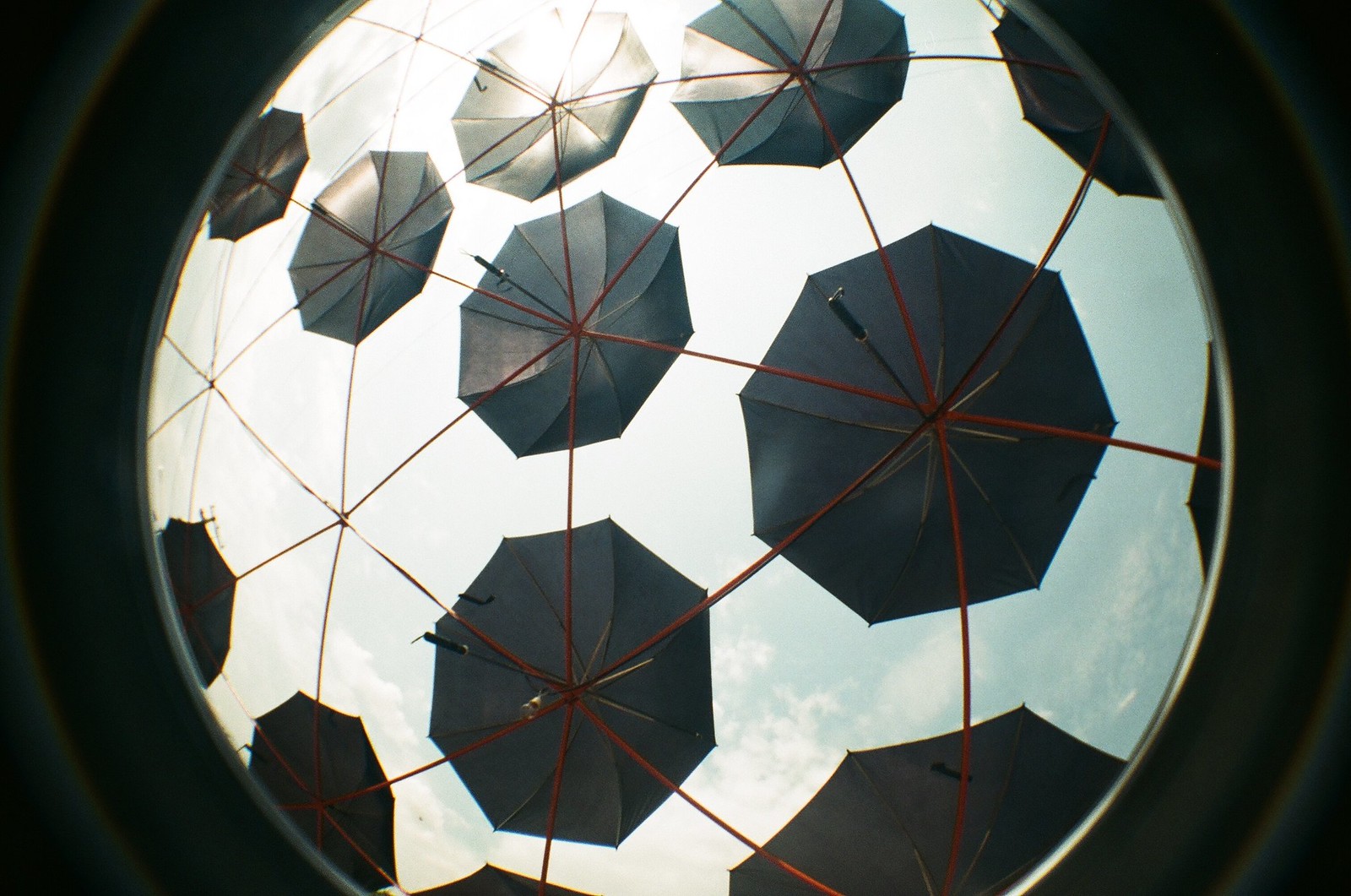This photograph features a creatively framed circular image within a rectangular border. The area outside the circle is black, giving the impression of a looking through a porthole or a fisheye lens without edge distortion. The viewer's perspective is from the bottom, looking upward through nearly a dozen identically black or dark gray umbrellas. These umbrellas are supported by a lattice of red, pyramid-like scaffolding, or possibly a wire mesh with brown lines intersecting at regular intervals. The sky above is a light blue, dotted with clouds, and sunlight filters through some umbrellas, creating a dramatic interplay of light and shadow. The handles of the umbrellas point downward, adding a unique geometric alignment to the scene.